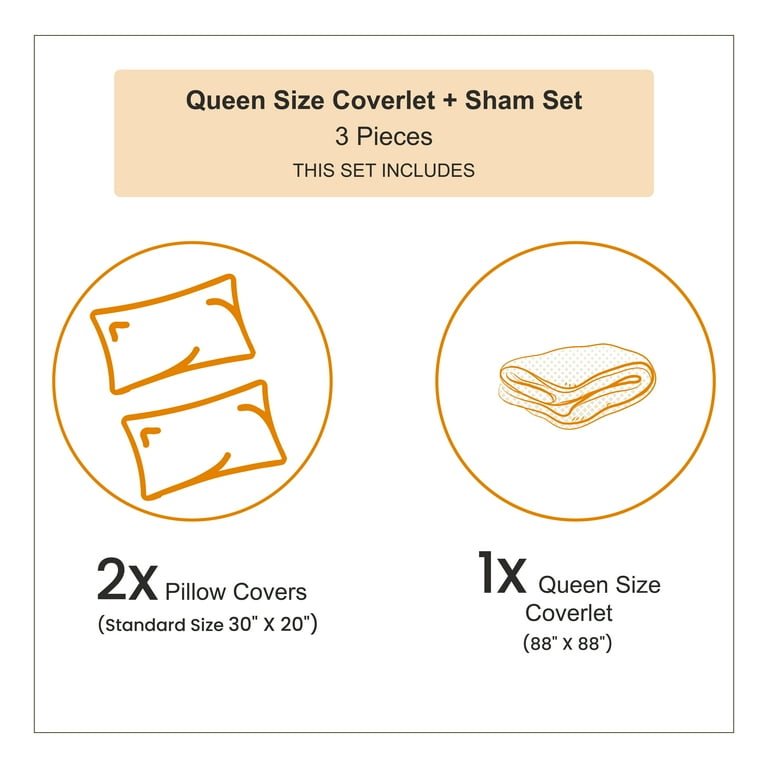The image is a vertically rectangular, three-color promotional instruction manual for a queen-size coverlet and sham set. It features a faint, thin black border and is predominantly white, matching the background of a computer screen. At the top, there is a horizontally rectangular pink (or peach) area with bold black text that reads, "Queen Size Coverlet Plus Sham Set – Three Pieces, This Set Includes."

Centrally, there are two gold (or orange) circles. The left circle contains an illustration of two gold (or orange) pillows, while the circle on the right shows a gold (or orange) folded coverlet. These images emphasize the set's contents. Below these circles, the left section has the text "2x Pillow Covers, Standard Size 30 inches by 20 inches," and the right section has "1x Queen Size Coverlet, 88 inches by 88 inches."

The illustrations and text are all simple and surrounded by a thin black line, ensuring they stand out clearly against the background.